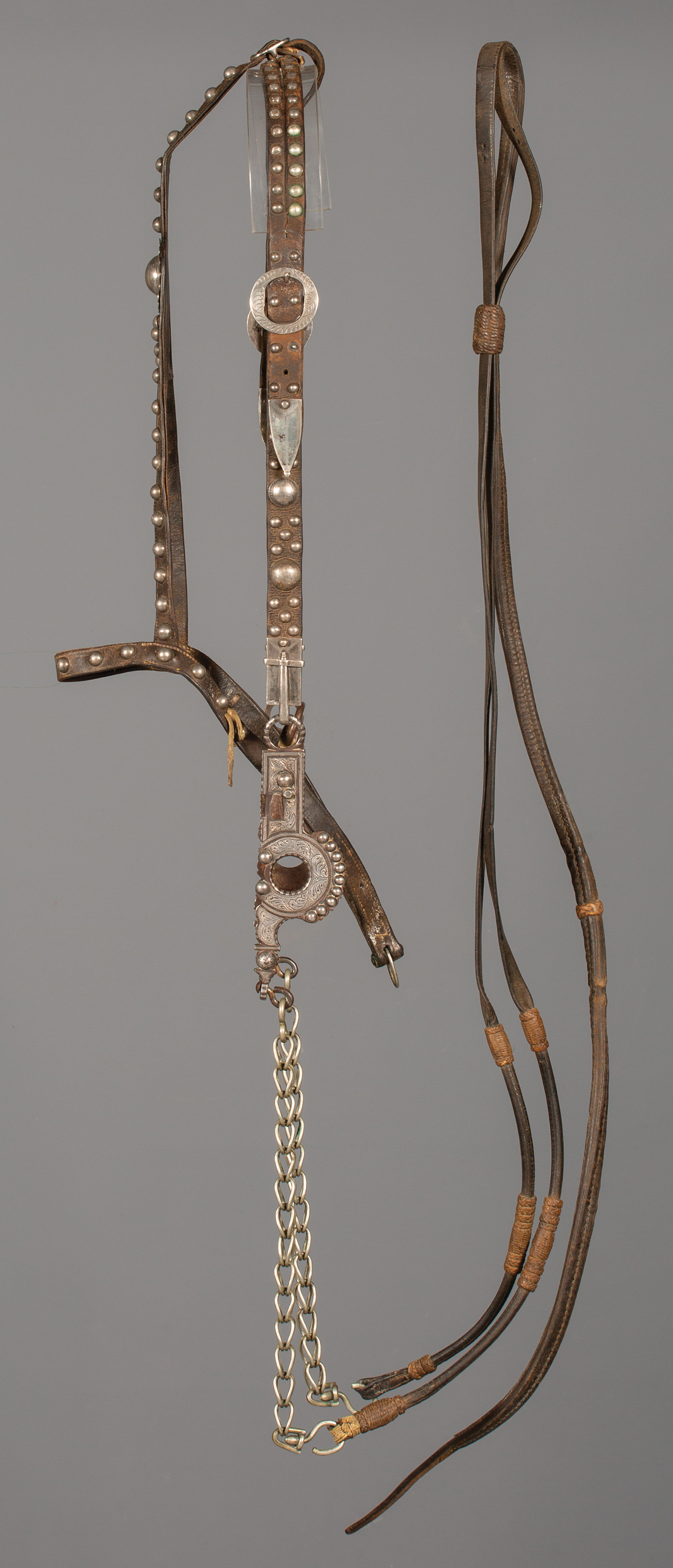The image depicts a detailed arrangement of horse equipment against a dark grey background. Central to the composition is a medium brown bridle adorned with gold studs, featuring a silver buckle and an elegant gold chain. The bridle is hanging on a clear plastic hook attached to the wall. Attached to the harness, which is crafted from brown leather, are reins interspersed with lighter brown beads, suggesting a decorative or functional element. These reins are strung between various wooden pegs, contributing to the intricate display of the horse tack. The overall appearance is suggestive of a carefully crafted, possibly high-end or ceremonial, equestrian accessory set, emphasized by the meticulous detailing and embellishments.